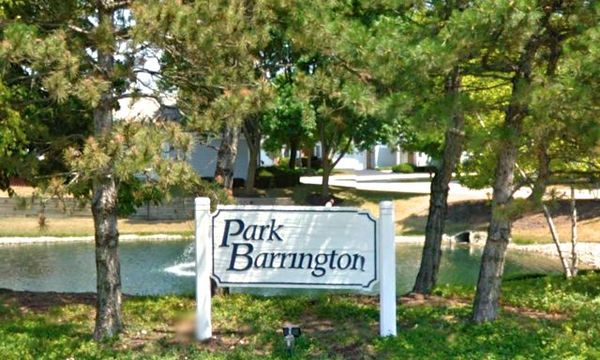The image depicts a scene from Park Barrington, as indicated by a prominent blue sign held by two white wooden posts. The rectangular sign, with angled corners and a blue trim, features the park's name in navy blue text slightly offset to the left. Below the sign, there are patches of green grass amidst a mostly sparse ground cover. In the background, there is a serene pond with a fountain, surrounded by numerous tall pine trees that provide a green backdrop. Bordering the pond, there's a strip of brown, dried grass. Beyond the pond, several light gray buildings, possibly homes or part of a business park, are visible, contributing to a picturesque and tranquil setting. A road winds its way toward the buildings and around the pond, completing the park-like ambiance.